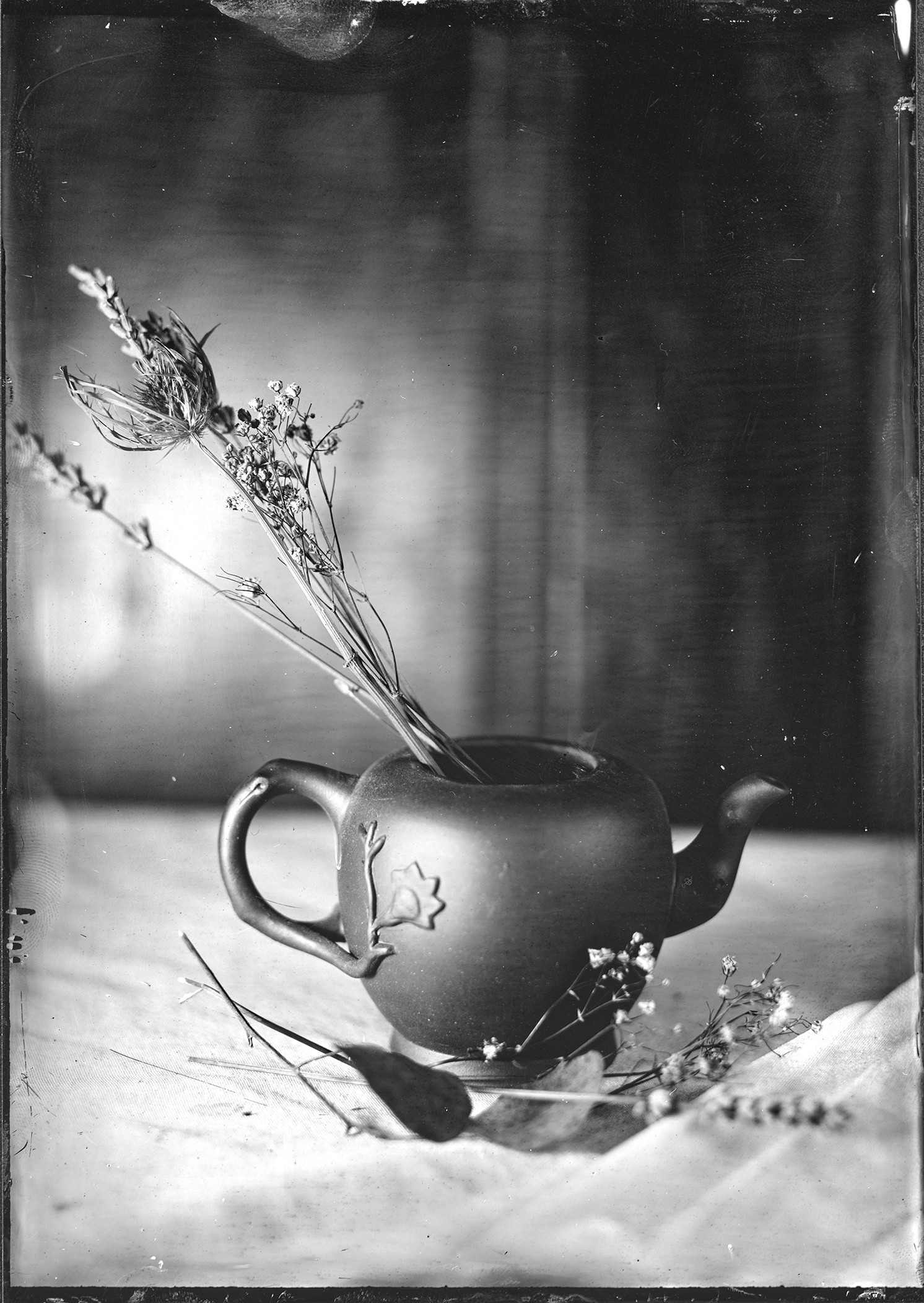This realistic, black and white photograph captures an antiquated ambiance through its aged filter and edited edges, which give it a vintage feel. The central focus is a teapot with a brushed metal finish and an elegant, raised flower design. The teapot, notably lidless, contains an arrangement of dried flowers and herbs, some of which spill onto the lighter-toned surface in front. The teapot’s handle and spout are distinctly visible, along with the etched floral details. The dried flowers, including a sprig of baby's breath, extend outwards, adding to the nostalgic essence of the scene. The blurred, dark background contrasts with the lighter foreground, emphasizing the teapot and its contents.